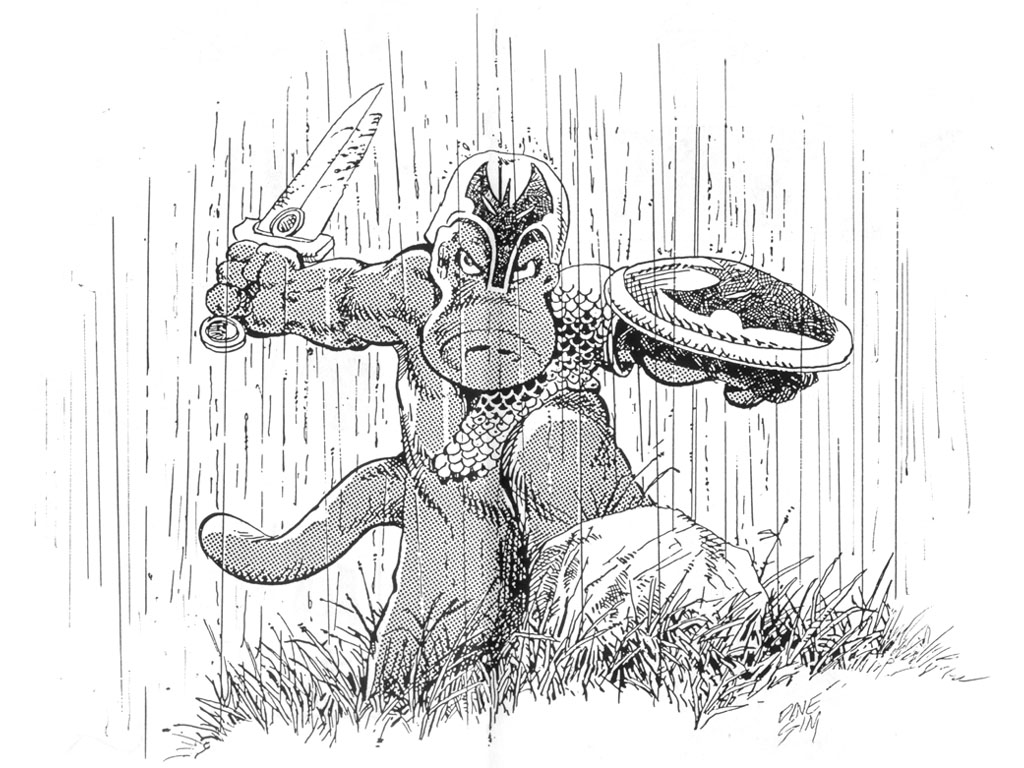This highly detailed, black and white pencil drawing depicts a fierce, warrior-like dinosaur character reminiscent of Bowser from Super Mario. The dinosaur, dressed in full battle gear, including armor on its chest and a menacing helmet, stands with a dagger in its right hand and a shield in its left. One of its feet is confidently perched on a rock, adding to its imposing presence. The detailed sketch includes lines that suggest rain falling across the outdoor scene, possibly indicating a daytime setting. The character's fierce expression and eyes convey readiness for battle. Additional elements include patches of grass around the rock and a barely legible signature by the artist. The entire drawing is composed of intricate lines and shading, focusing on the dynamic and intense portrayal of this warrior dinosaur.